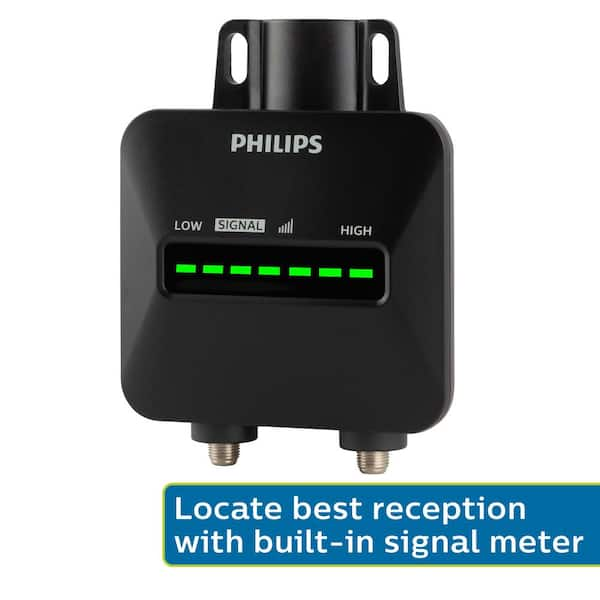The image depicts a black square-shaped device against a white background, branded with the name "Philips" in capital white letters at the top. The device appears to be some sort of signal detection or antenna equipment, designed to gauge signal strength. It features two handles or attachment points on top and two coaxial cable-like receptor posts at the bottom.

In the center of the device, there is a series of seven green LED bars that indicate signal strength, with labels "LOW SIGNAL" on the left and "HIGH" on the right, both in capital letters. The bottom of the device has a blue border with white text that reads, "Locate best reception with built-in signal meter." This suggests that the device aids in finding optimal signal strength, possibly for Wi-Fi or some form of connectivity.